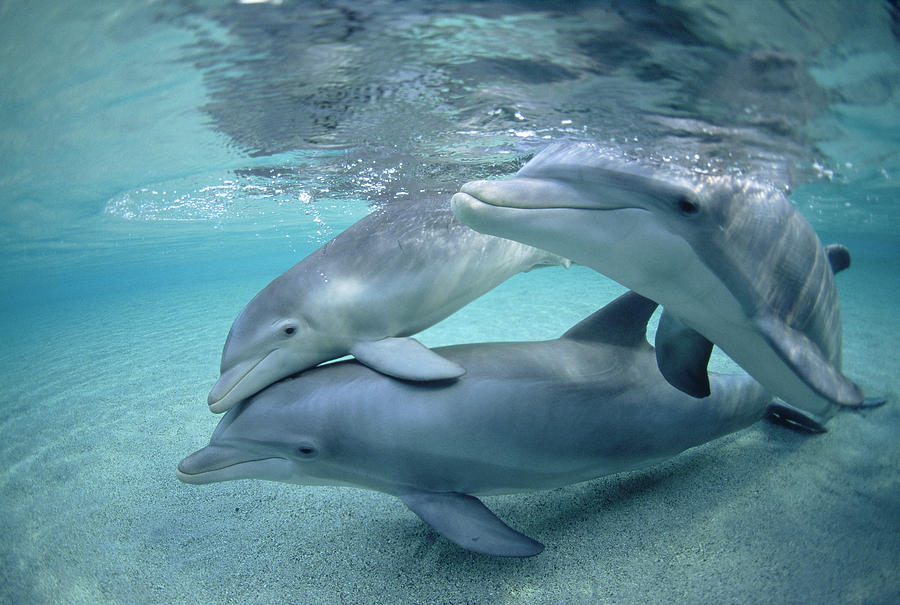The image captures a vibrant underwater scene with three gray dolphins, characterized by their white underbellies and streamlined bodies, swimming through shallow, greenish-blue water. All three dolphins have closed mouths and small, black eyes, and their faces are oriented to the left. The dolphin at the bottom of the frame is in contact with the sandy pool floor, while a smaller dolphin above it appears to be resting its fin on the one below. The third dolphin, positioned to the right, seems to be moving towards the camera, with the top of its head breaking the surface of the water. Above the dolphins, the water has a cloudy, grayish-green hue, and the reflections of the dolphins are visible on this turbulent water surface. The scene is set against a backdrop of clear, plant-free sand.